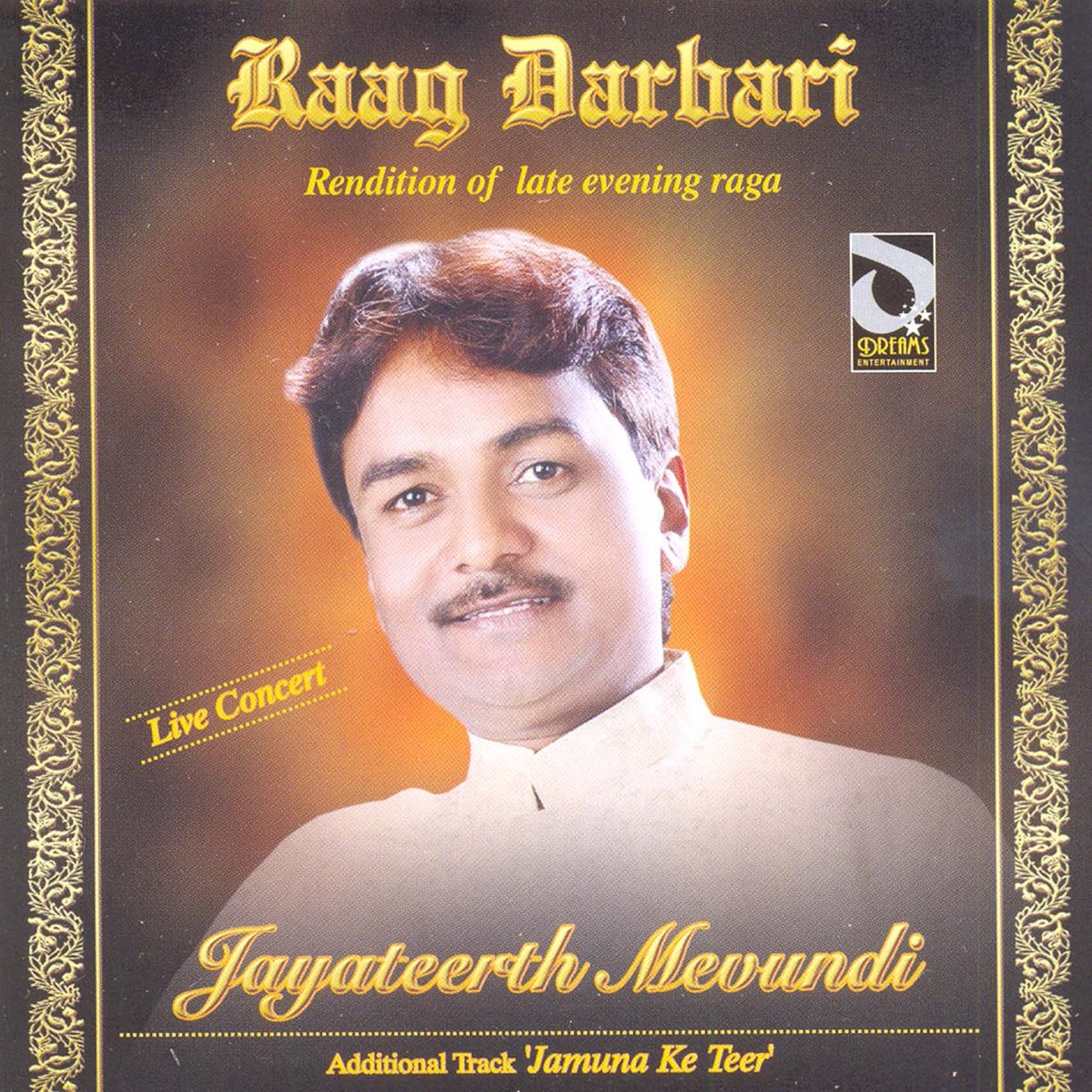The CD cover features a young Indian artist, likely in his late 20s or early 30s, with wavy, dark brown hair and a brown mustache, dressed in a white, stiff-collared shirt. The artist's name, Jayatirth Mevundi, is displayed in elegant yellow cursive text. The title "Raag Darbari" is prominently positioned at the top in a bold, yellowish-gold gradient font. Beneath it, in smaller yellow text, it states "rendition of Late Evening Raga." The words "Live Concert" appear to the left of the artist's face in small yellow text. Additionally, there is a mention of an "additional track: Jamuna Khatir" in smaller yellow text below a dotted horizontal line. The left and right sides of the cover are adorned with an embossed gold border featuring intricate, filigree-like Indian cultural designs.